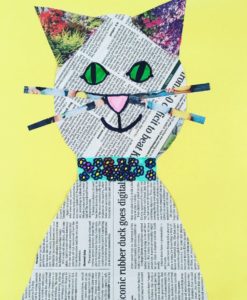The image shows an amateur yet vibrant rectangular collage of a cat, facing the viewer, crafted from newspaper print. Centered against a bright yellow background, the cat captivates with its collage details. Its pink nose and vividly green eyes with black pupils draw immediate attention. The cat's whiskers, also fashioned from newspaper snippets, add a whimsical touch. Its ears, resembling colorful birthday party hats, are a mix of green, red, purple, and pink hues, integrating floral patterns. The cat sports a multi-hued collar, primarily blue and black, that contrasts with its newspaper-textured body. The scattered readable text, including phrases like "This iconic rubber duck goes digital," adds a layer of intrigue. Despite its simplistic appearance, the detailed and brightly colored elements suggest a playful and imaginative piece, perhaps created for sheer fun.